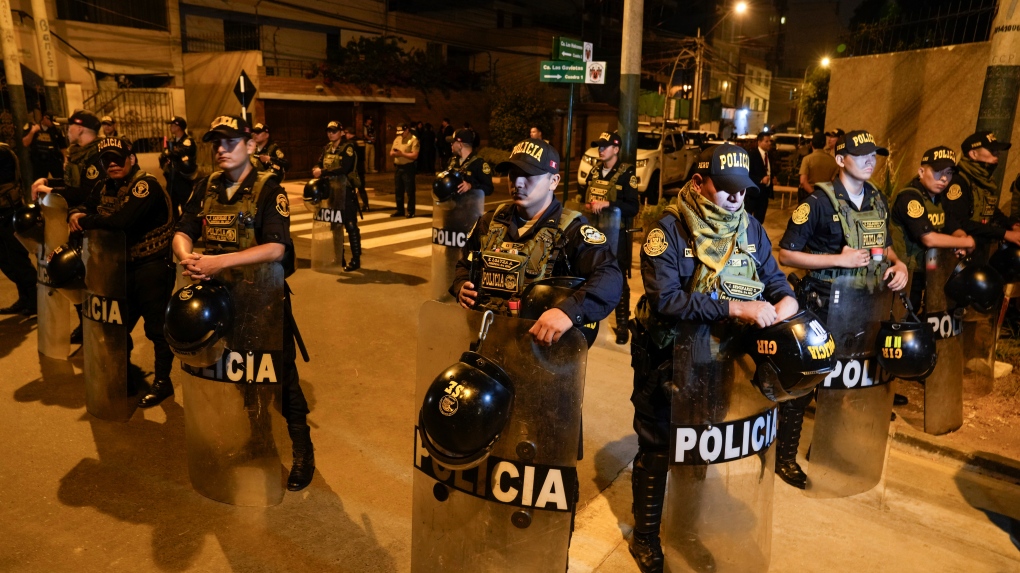The image depicts a large, long, rectangular urban scene bathed in brassy gold tones, evoking a menacing atmosphere. It's nighttime, the dark sky revealing scattered buildings in the far distance, central to the composition. Foregrounded is a street, identifiable by its white markings, flanked by wooden structures to the right and left. A notable black pole topped with wood stands prominently in the middle, accompanied by distant streetlights and a black pole adorned with green signs.

At the heart of this scene is a formidable formation of police officers, branded "POLICIA" in bold white letters across their clear, large riot shields. Their numbers suggest a state of high readiness, seemingly prepared to handle a potential riot. Positioned strategically, four officers are on the right, three on the far left, and one at the forefront, with others visible in the background. Dressed in navy blue uniforms accented by green or yellow bandanas, vests, white epaulettes, and blue caps featuring the word "POLICIA" in yellow, they present a uniformed front. Their serious facial expressions, some with sunglasses, add to the tension, conveying a no-nonsense readiness for duty.